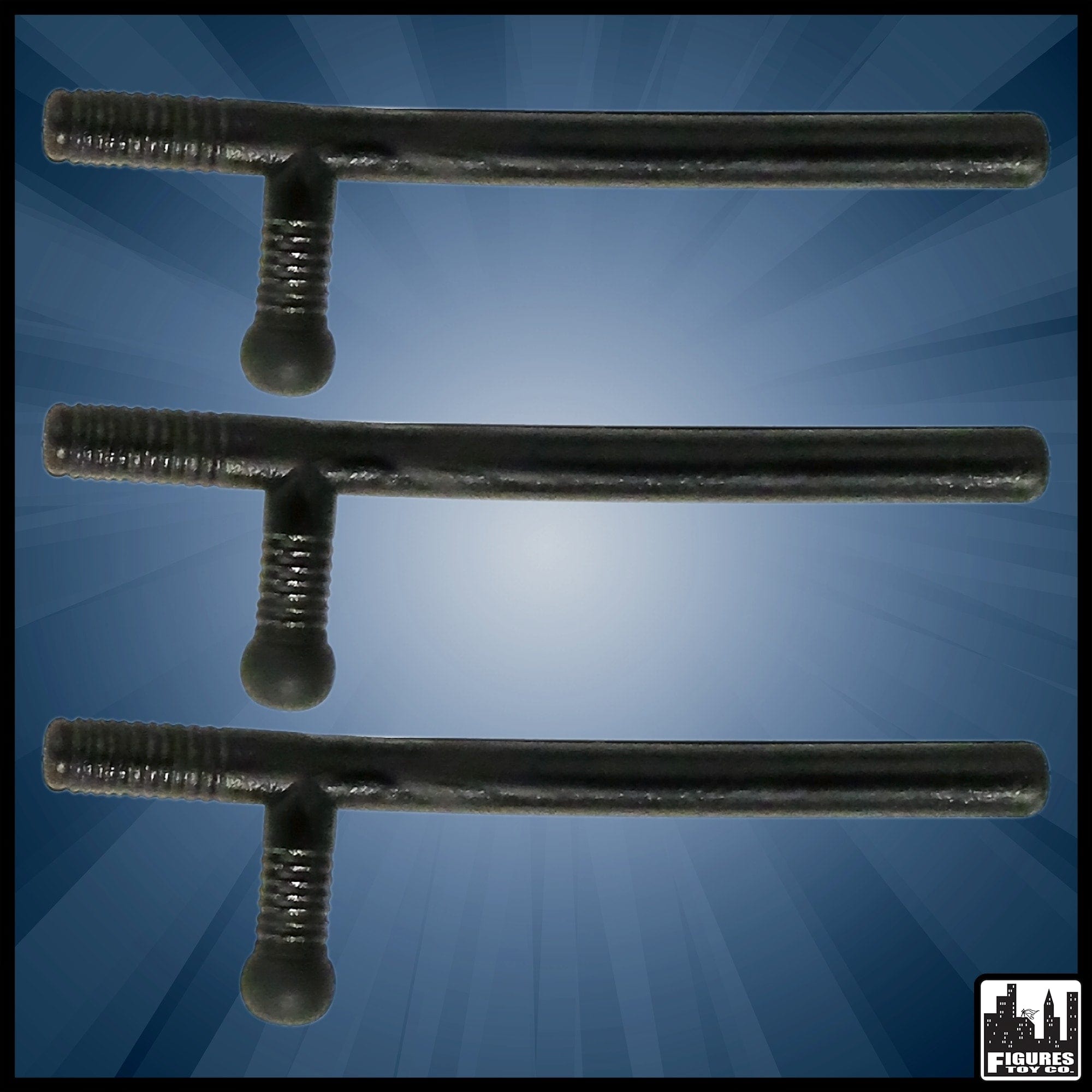This photographic image features three black pieces of equipment prominently displayed against a blue background with a radiant white light at the center, dispersing beams like sun rays. The equipment consists of batons that have a handle perpendicular to the main shaft, resembling martial arts tonfas or riot police batons. These batons are shiny, possibly made from wood or metal, with ribbed handles for better grip, and are lined up horizontally with the handles positioned to the left. There is no writing on the batons themselves. In the bottom right corner of the image, there is a square logo with a black city skyline graphic and the text "Figures Toy Company."